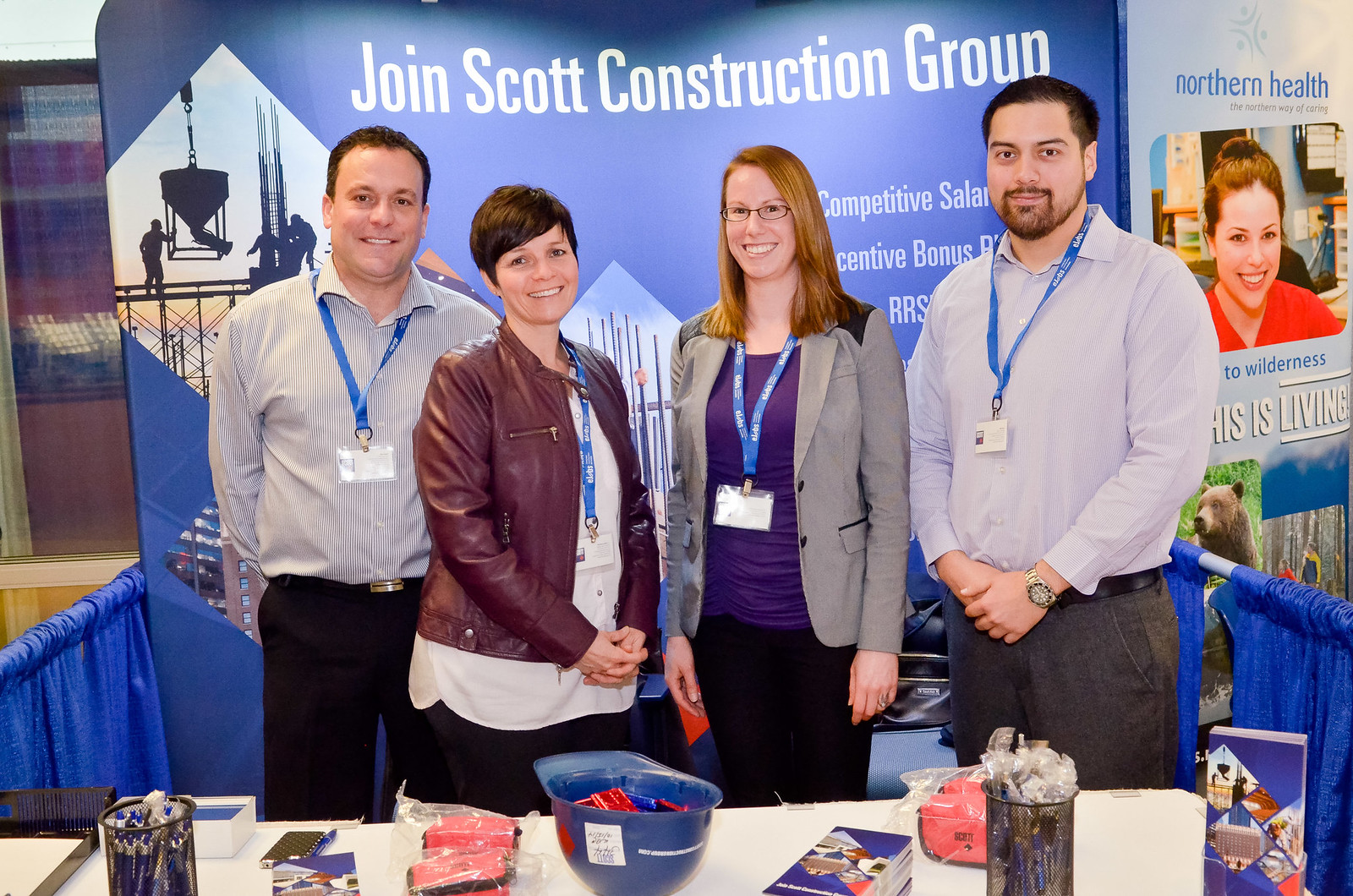In this photographic image, taken indoors at an expo hall, four individuals—two men and two women—pose in front of an exhibit table. Behind them is a prominent blue banner that reads, "Join Scott Construction Group: Competitive Salaries, Incentive Bonus," featuring an image of workers lowering a heavy bucket from a crane. The man on the left is dressed in a gray striped shirt and black pants, next to him is a woman in a brown leather jacket, white shirt, and black pants. Beside her stands another woman in a gray jacket, purple shirt, and black pants, followed by a man in a gray shirt, black pants, and a wristwatch. Each person sports a blue lanyard with a name tag. 

In front of them, the white table is laden with typical convention giveaways: an upside-down blue construction helmet with something inside, two canisters likely filled with pens, packets of small wallets, and various brochures. The setting features additional exhibit areas, including one to the right with a sign reading, "Northern Health Wilderness, This is Living." The backdrop includes metallic poles supporting blue carpet curtains.